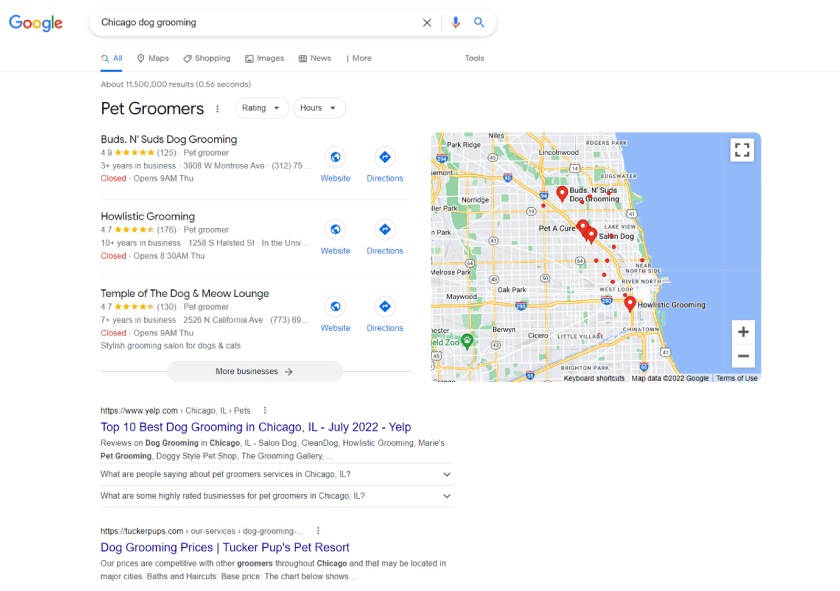Displayed on Google's homepage, the search query is centered around "dog grooming." Positioned approximately two inches from the left edge, the Google logo features its classic multi-colored design in the top left corner. Directly underneath and spanning halfway across the page is a prominent search bar containing the text "dog grooming" in black font. To the right of the search bar, there are three icons: an "X" for clearing the search, a microphone for voice search, and a magnifying glass for executing the search.

Below the search bar, a blue-highlighted "All" option appears, indicating the active search category, flanked by several other options—"Maps," "Shopping," "Images," "News," and "More"—each accompanied by an icon on their left. Further to the right, there is an option labeled "Tools."

Beneath this menu, the number of search results and the time taken to retrieve them are displayed. Following this, the heading "Pet Groomers" appears in bold letters. Below, two white tabs with black lettering are visible: one labeled "Rating" and the other "Hours."

The search results list three dog grooming businesses, each entry displaying the name of the business, their star rating, the number of years in operation, and the address. Adjacent to this, the business hours are listed on the right side, with links to the website and directions provided.

A map occupies the right third of the screen, wherein the right portion depicts blue water and the remainder, a mix of tan and green areas marked by yellow lines. Four red pins are distributed mostly in the central region of the map.

On the left side, a small gray tab with the text "More businesses" in black and an arrow pointing to the right is shown. Beneath the main search results, there are two additional clickable links.